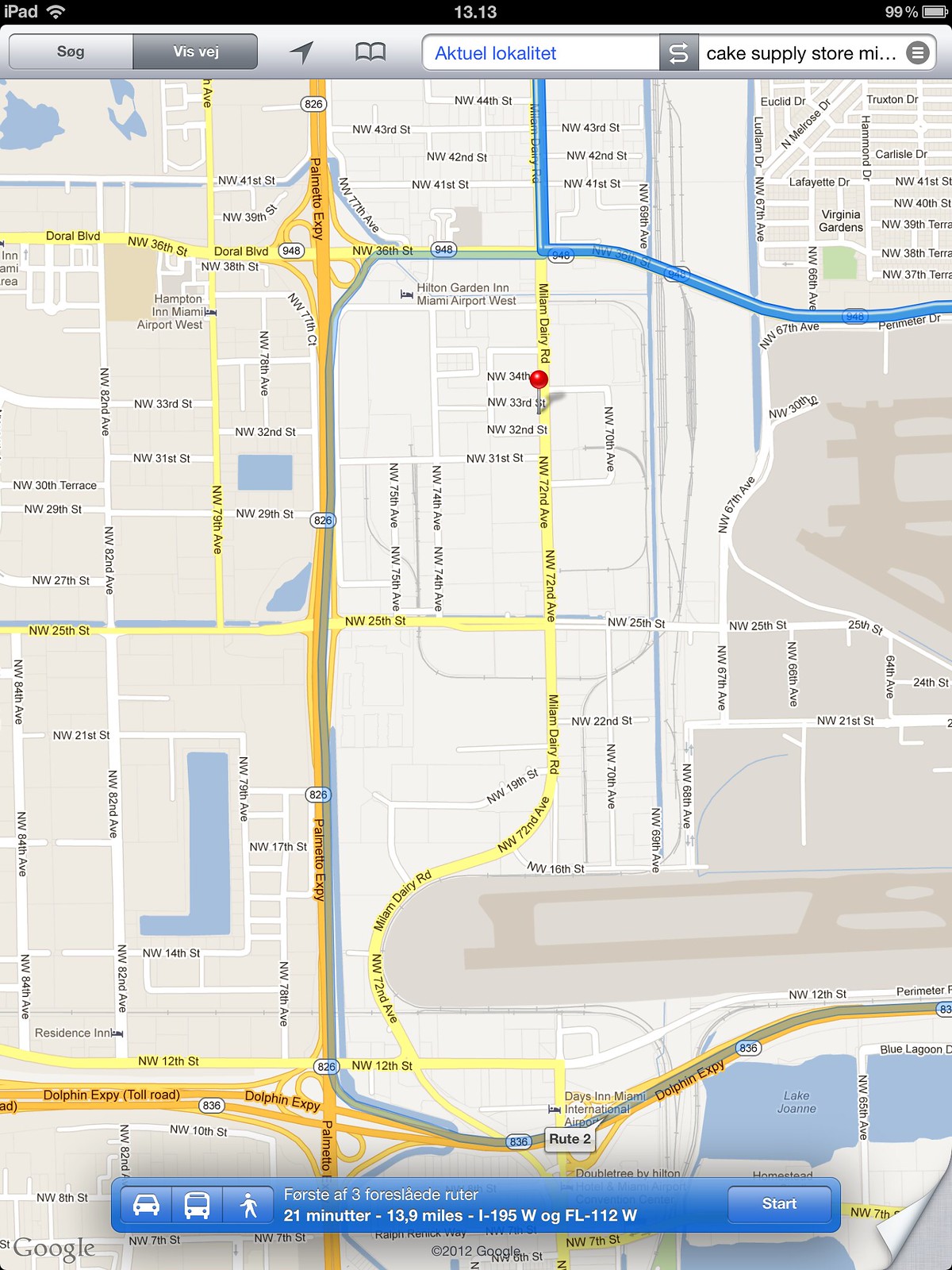A detailed screen capture from a map application displayed on an iPad showcases various urban streets arranged in a horizontal and vertical grid. At the top of the image, a ribbon interface shows "iPad" on the upper left, "13.3" in white lettering centered, and "99% power" to the upper right. Below this ribbon is a search bar slightly right of center containing the text "AKTUELL OKALITET" and, to its right, "Cake Supply Store MI."

At the bottom of the image, a minimal overlay features three icons to the left, followed by partially obscured text. Below this, the display reads "20 minutes - 13 miles," followed by route information "I-195 West OGF L112 W," and to the right is a prominent "Start" button.

The central portion of the image depicts a detailed collection of numbered and lettered streets. A major highway, denoted as "806," runs vertically from the top to the bottom, slightly left of center. The background features a largely tan color scheme, with a distinct darker tan area on the right, likely indicating an airport field.